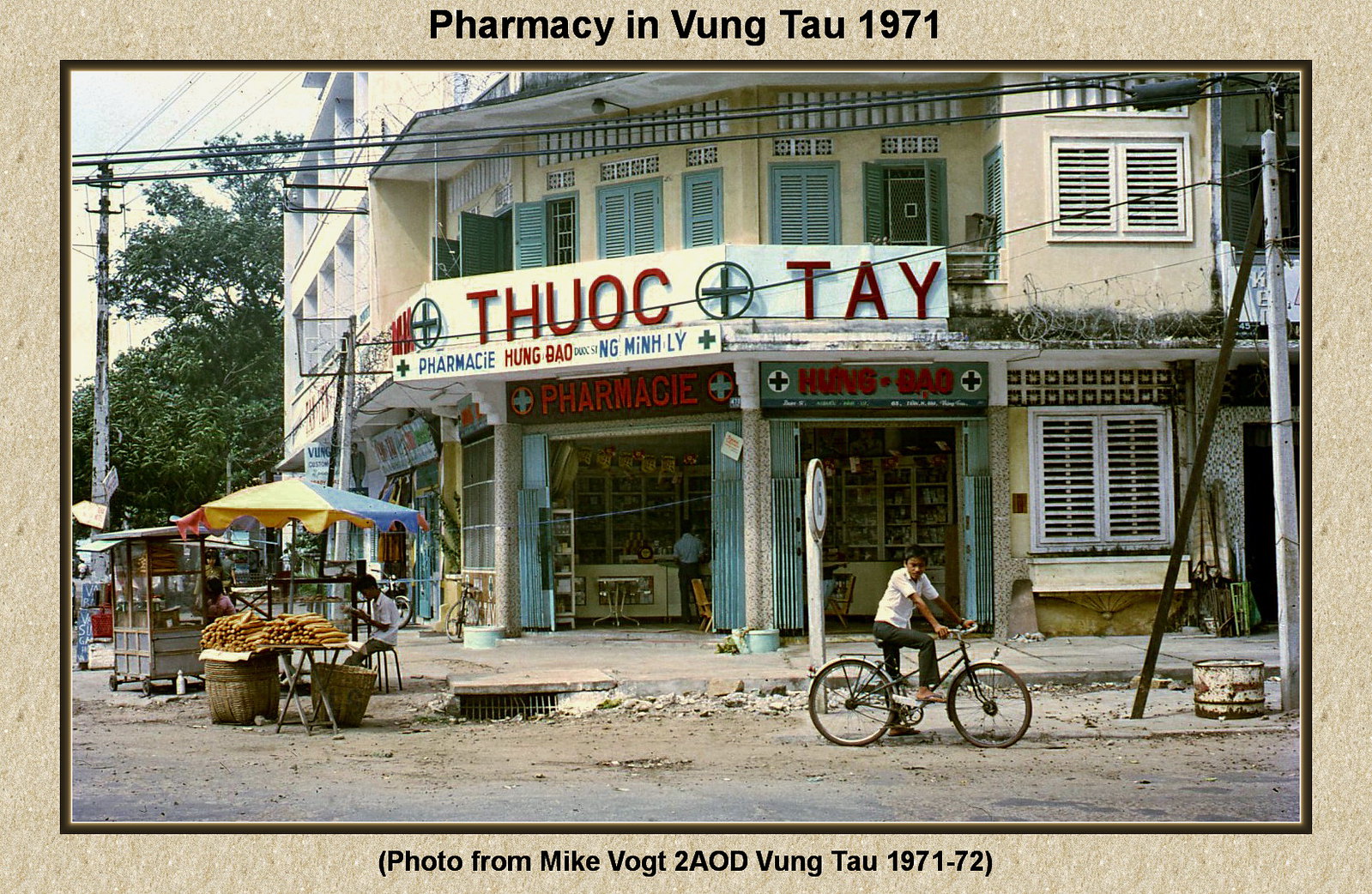In this image, a historical photograph with a tan border features prominently. The border includes text that reads, "Pharmacy in Vung Tau, 1971. Photo from Mike Vogue, 2 AOD Vung Tau, 1971-72." Captured in the bustling streets of Vung Tau, Vietnam, the scene depicts a dilapidated street with evident signs of wear and decay. A man rides a bicycle through the scene, while various street vendors can be seen engaging in their daily activities. Centrally located within the image is the entrance to a pharmacy. The photograph is rich in colors, notably tan, black, white, blue, red, yellow, gray, and black, illustrating the vibrant yet worn nature of the setting. The snapshot appears to capture an outdoor environment bathed in daylight, offering a poignant glimpse into a moment of everyday life in Vietnam during the early 1970s.